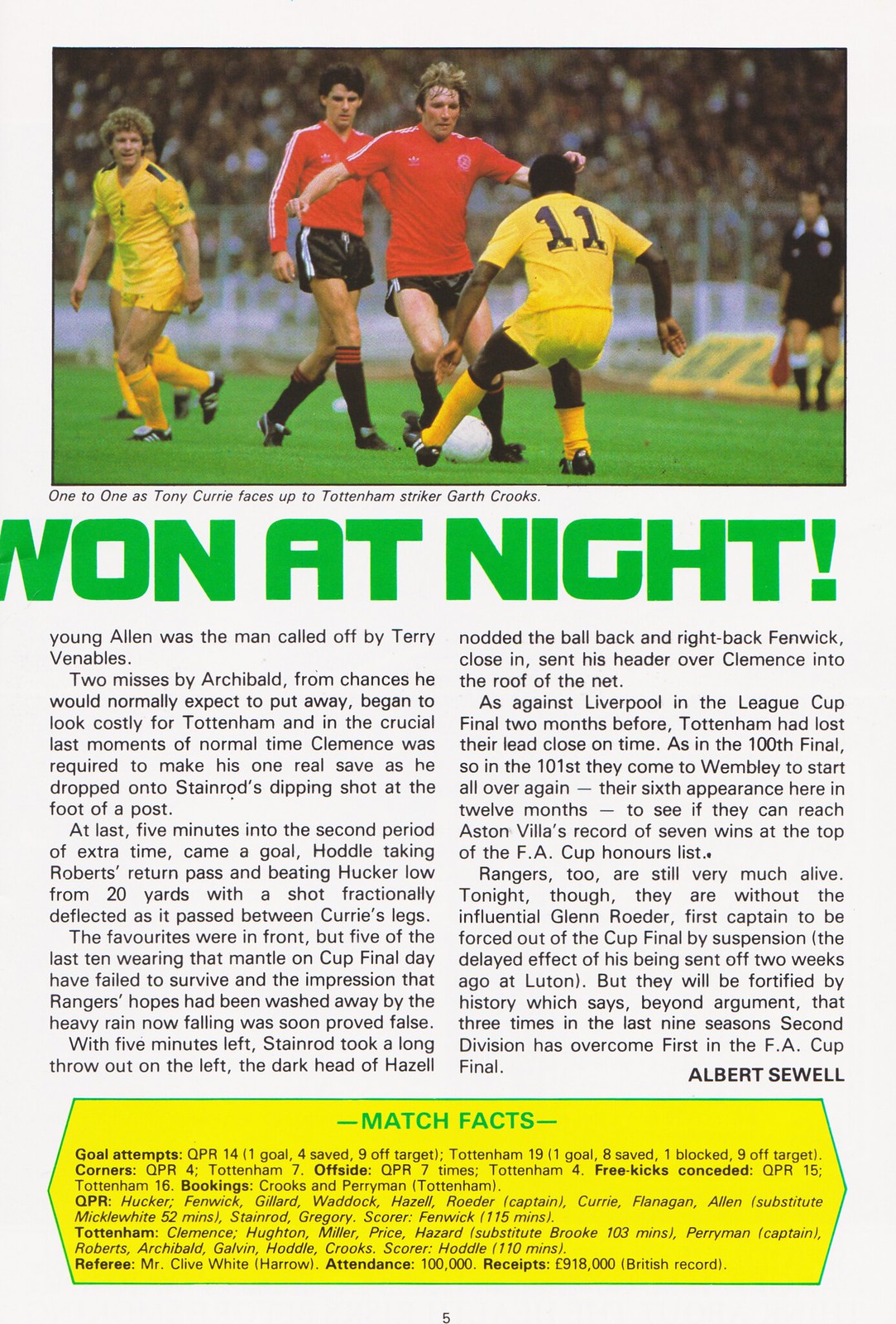The image depicts a page from a sports magazine, specifically a detailed soccer program. The top third of the page features a vibrant, landscape-oriented photograph capturing five players in action on a lush green field. Two players, donning red jerseys and black shorts, are engaged with three players who wear yellow jerseys, shorts, and socks. One red-jerseyed player is poised to kick the white soccer ball, while a yellow-jerseyed player, with the number 11 on his back, is seen tackling him from behind. In the distant background, a referee clad in black holds a red flag. Blurred spectators in the stands and various sponsor billboards line the stadium perimeter.

Beneath the photograph is a bold headline in all caps, "ONE AT NIGHT." Following this, the article, authored by Albert Sewell, details an intense match between Tottenham Hotspur and Queens Park Rangers (QPR). The narrative recounts key moments, including missed opportunities, a late goal by Hoddle, and an eventual comeback by QPR, leading to a dramatic finish.

At the bottom of the page, the page number 5 is centered, flanked by a yellow box with green borders, serving as a statistical summary labeled "Match Facts." The box provides detailed game statistics, including goal attempts, corners, offsides, and individual bookings for players. The detailed stats indicate a closely contested match, highlighting the intensity and competitiveness of the game. The entire depiction encapsulates the energy and details of a captivating football match, making the page an informative and engaging read for soccer enthusiasts.